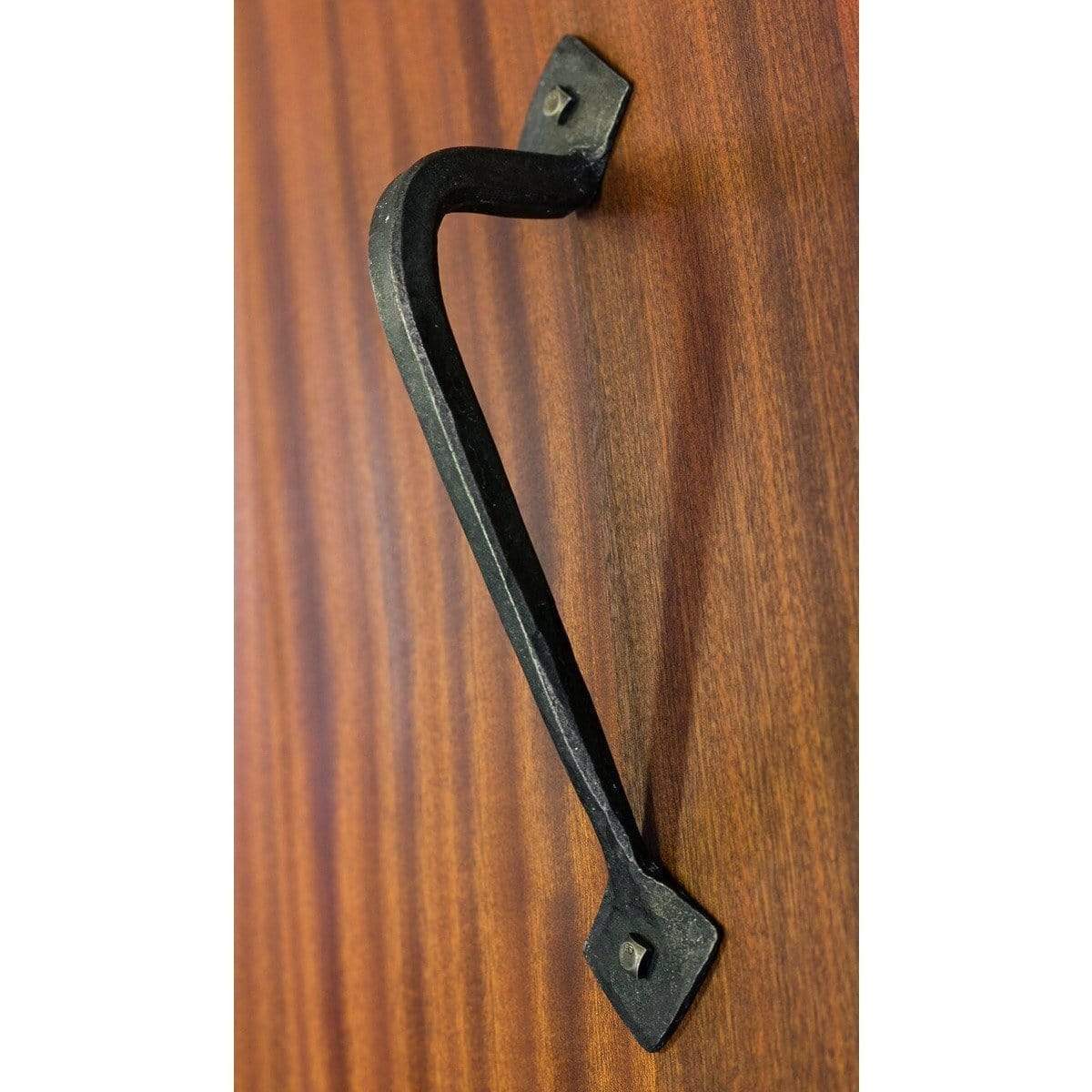This color photograph captures a rustic iron door handle securely bolted onto a dark brown wooden surface. The handle, crafted from dark metallic iron, features an upward curving design that begins low at the bottom, extends outward, and loops back at the top. Both ends of the handle form diamond shapes, each fastened to the wood with a small, steel-colored screw, enhancing its antique aesthetics. The wooden background showcases a visible grain with grooves of a deeper brown running vertically. The handle casts a distinct shadow upon the wood, adding depth and dimension to the portrait-style image. There are no human, animal, or other structural elements present in the photograph, emphasizing the simplicity and texture of the handle and wooden surface.